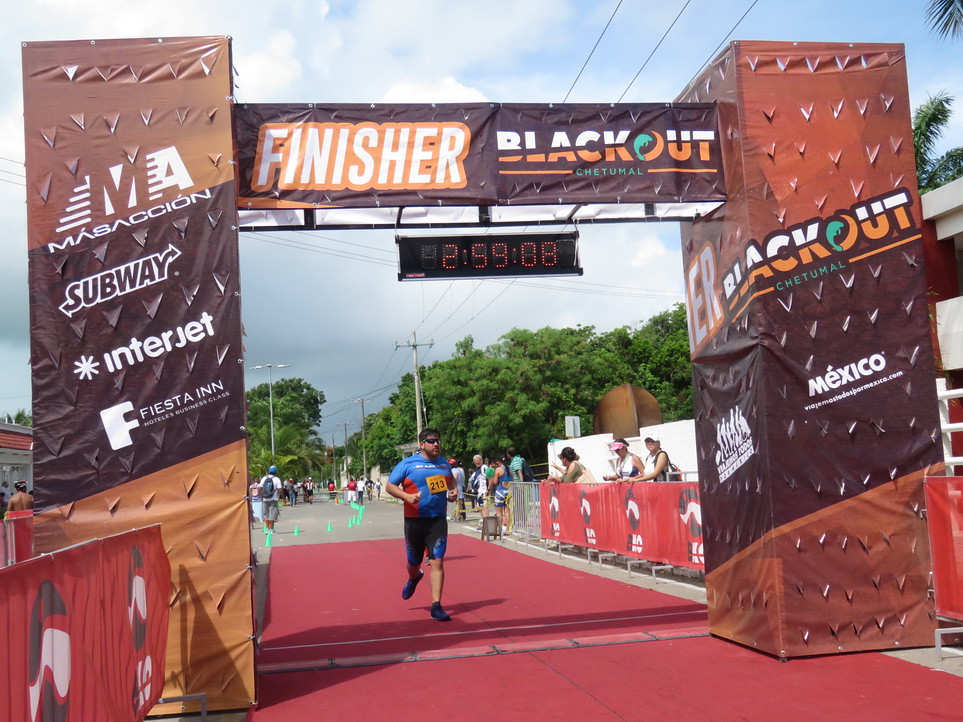In this compelling image of the final moments of a marathon, we witness a muscular runner crossing an outdoor finish line under a digital clock displaying 2 hours, 59 minutes, and 8 seconds. The finish line is marked by a banner adorned in different shades of brown, inscribed with "Finisher, Blackout Chetumal." Standing out beneath this banner are two square posts covered in various logos, including ABS2, M-E-M-A-S-A-C-I-O-N, Subway, Interjet, Fiesta Inn, Hotels, and Business Class, with a mention of Mexico. The runner, sporting a blue and red shirt with the number 213 on a yellow bib, dark sunglasses, black and blue shorts, and blue sneakers, pushes through the final steps on a red carpeted pathway. Flanking him on both sides are enthusiastic spectators behind red barriers, cheering him on against a backdrop of distant trees and a cloudy sky. His solid build and determination are evident as he powers through nearly three hours of relentless effort.